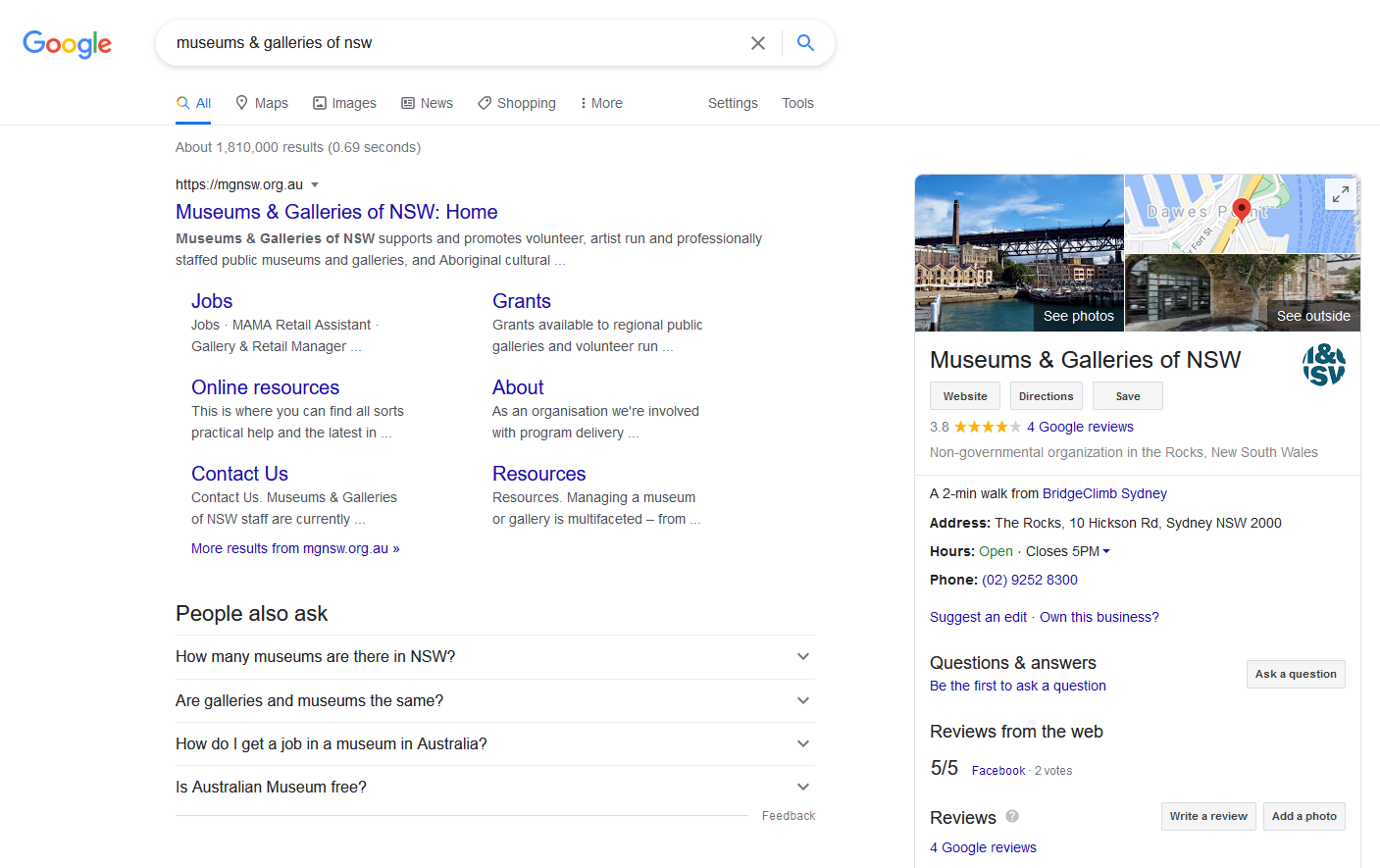This image is a detailed screenshot of a Google search engine results page. The background color is a clean white, and positioned in the upper-left corner is the iconic Google logo, featuring the familiar sequence of a blue 'G', red 'O', yellow 'O', blue 'G', green 'L', and red 'E'. To the right of the logo is the search bar, containing the query: "museums and galleries of NSW".

Below the search bar, the primary search result is for "Museums & Galleries of NSW", with the homepage URL "mgnsw.org.au" indicating it is an Australian website. Beneath this main listing, various categories are available, including "Jobs", "Online Resources", "Contact Us", "Grants", "About", and "Resources".

In the upper-right corner of the search results page, there is a detailed listing for "Museums & Galleries of NSW". This section features two photos and a portion of a map. Dominating this section is the bold, black text "Museums and Galleries of NSW", followed by a user rating of 3.8 stars, visualized with gold stars. Also displayed are buttons for easy navigation to the website, getting directions, and saving the listing.